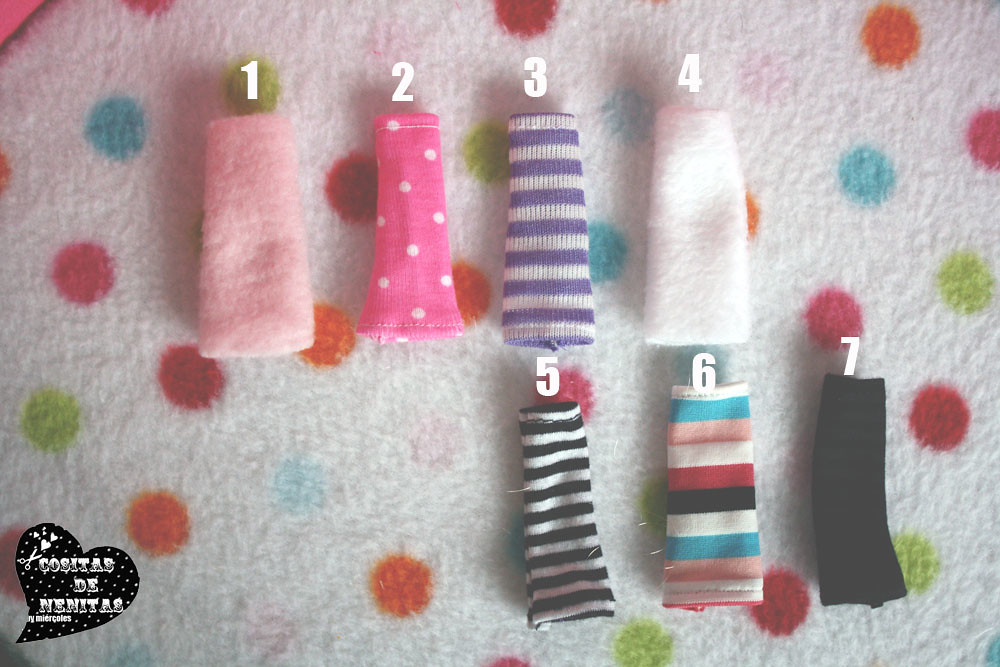The image features a white background adorned with colorful polka dots in red, blue, orange, green, and pink, reminiscent of a soft baby blanket or wool material. Spread out on this background are seven numbered fabric samples (1 through 7), each rectangular with an elastic end, possibly suggesting they are armbands or similar small textile items. 

The samples are arranged with four on the upper portion and three on the lower right side. From left to right in the upper row: number 1 is a soft light pink, number 2 is a dark pink with white polka dots, number 3 is gray and purple horizontal stripes, and number 4 is pure white. On the lower right side: number 5 features black and white horizontal stripes, number 6 is a multicolored striped pattern including hues of white, turquoise, peach, red, black, and pink, and number 7 is plain black. In the bottom left corner of the image, there is an overlay of a black heart logo with white lettering that reads "Cositas de Netas," accompanied by white circles and scissors.